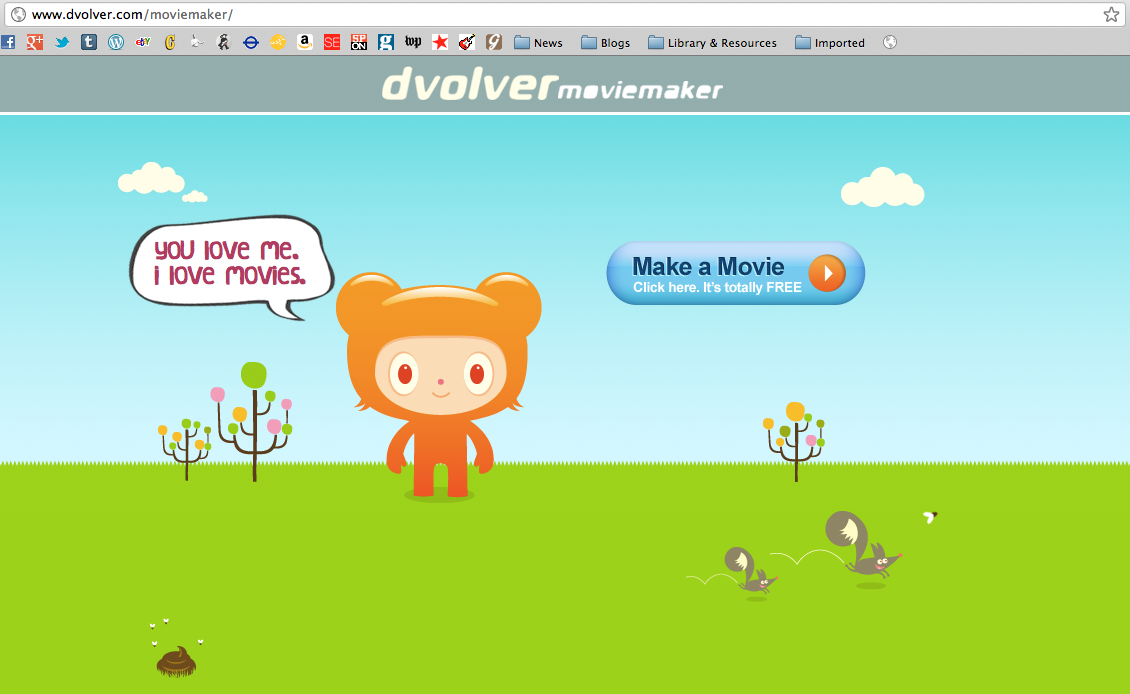The image is a screenshot of a website, displaying various UI elements and whimsical graphics. At the top of the screenshot, a thin white rectangle denotes the search bar, containing the URL: www.devolver.com/moviemaker. Just below the search bar, a grey horizontal banner features folders labeled 'News,' 'Blogs,' 'Library & Resources,' and 'Imported,' along with icons for popular websites such as Facebook, Twitter, Tumblr, Amazon, and The Washington Post.

Under the banner, another grey bar displays the title "Devolver" in light yellow font with the subtitle "Movie Maker" in smaller white font. Below this, the main content of the webpage is presented.

The primary image showcases a vibrant scene featuring a lush green grass field and a turquoise sky adorned with a few small clouds. Central to the scene is an orange, bear-like creature with a text bubble that says, "You love me, I love movies." The webpage invites users to interact with a prominent blue rounded button that reads, "Make a movie, click here, it's totally free." Surrounding the cheerful bear-like creature are several cartoon squirrels, various trees, and a rather humorously placed pile of poop, adding a quirky touch to the overall playful aesthetic.